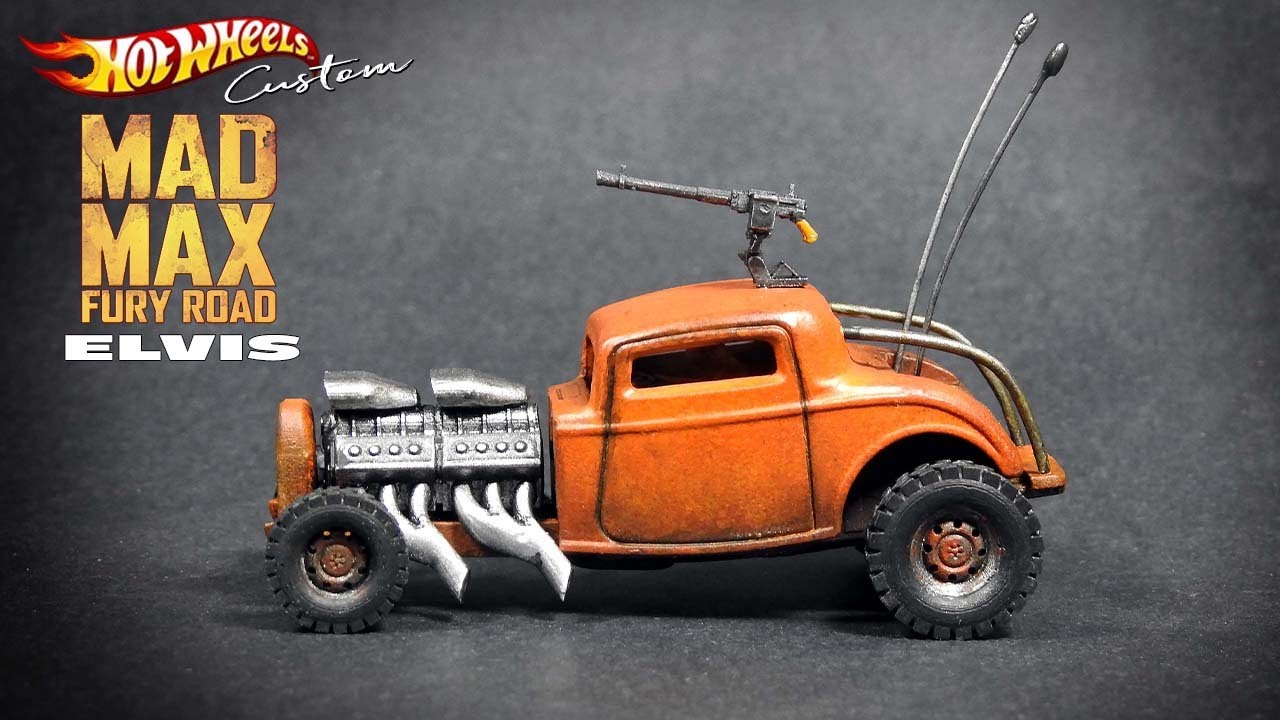The advertisement features a Hot Wheels Custom Mad Max Fury Road Elvis vehicle, set against a gray backdrop with a vertical orientation. In the top left corner, the iconic Hot Wheels logo is displayed in yellow with a red background and flames emerging from the large 'H'. Below this, the word "Custom" is written in white cursive, followed by "MAD MAX" in bold capital letters, "Fury Road" in smaller letters, and "ELVIS" in large capital letters beneath it.

The vehicle itself is an orange, roadster-type car with a heavily modified body featuring a prominent metallic engine that is uncovered. The engine appears to be a twin setup with intake and exhaust pipes conspicuously running out towards the bottom. The car has a distinctive look with its big rear tires and smaller front tires, indicative of a "funny car" design. A machine gun is mounted on the roof, alongside two silver antennas that extend from the back. The car's design includes a roll cage-like structure on the rear with two handrails extending from the roof to the bumper, providing a rugged, post-apocalyptic aesthetic. The overall presentation emphasizes the car’s unique and aggressive styling, suitable for the Mad Max theme.